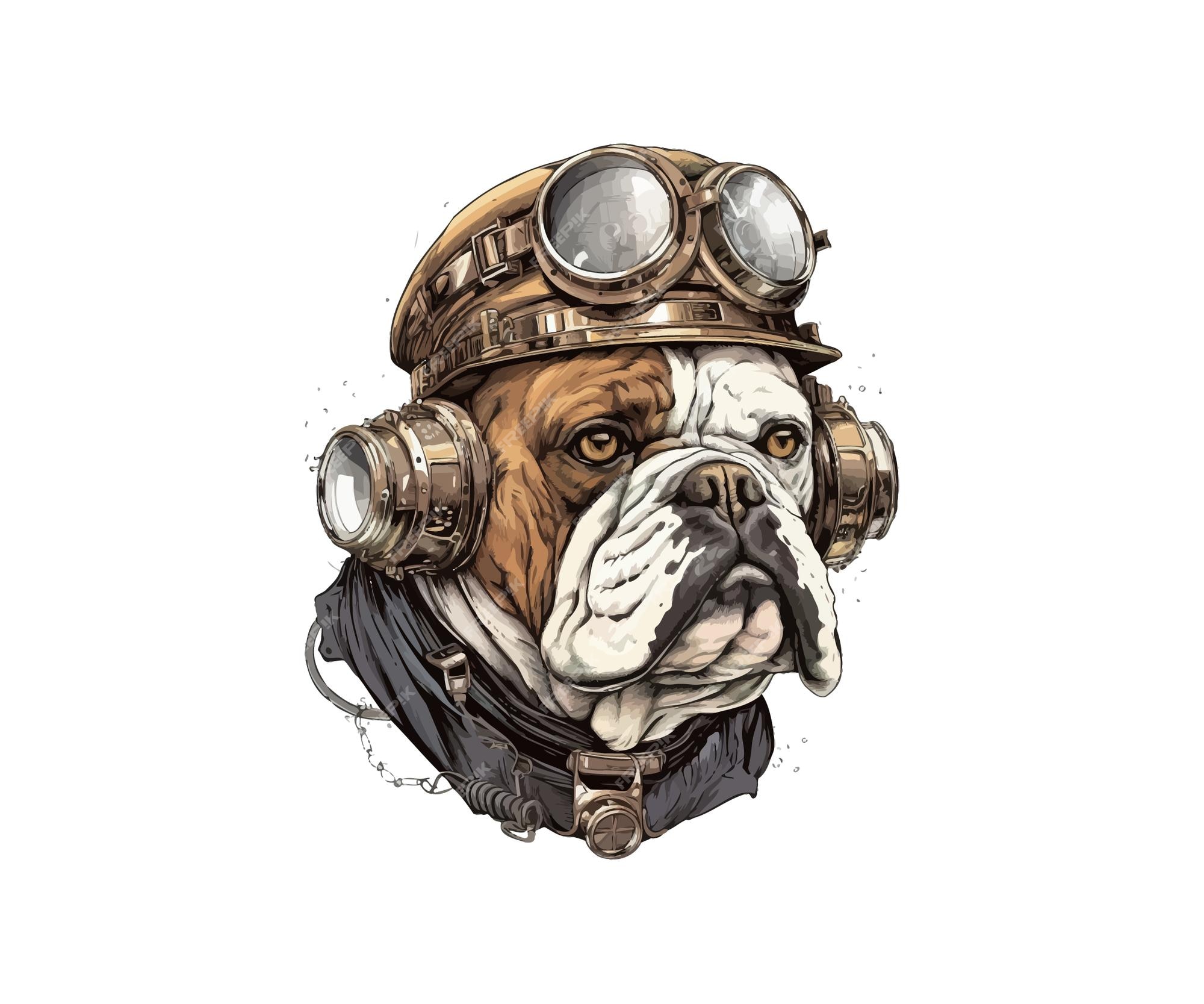This detailed digital illustration portrays an English Bulldog's head, exuding a playful yet focused demeanor. The dog's characteristic loose, wrinkled skin and prominent jowls are meticulously rendered, highlighting its breed-specific features. Its coat is predominantly white, with notable black markings around its lips and a distinctive brown spot gracing the left side of its head.

Adding to its charm, the bulldog is whimsically dressed in aviator attire. Atop its head rests a brown pilot's cap, accentuated with a brass-colored headband and a small bill. The cap is adorned with a pair of brown round goggles, enhancing the pilot theme. Flanking either side of the dog's head are what appear to be vintage headphones, contributing to the steampunk aesthetic.

The neck area features a scarf draped around it, detailed with metallic devices and chains, adding to the intricate design. The entire image is set against a stark white background, further emphasizing the central figure. Sparse black dots around the dog add a subtle, unfinished touch to the illustration.